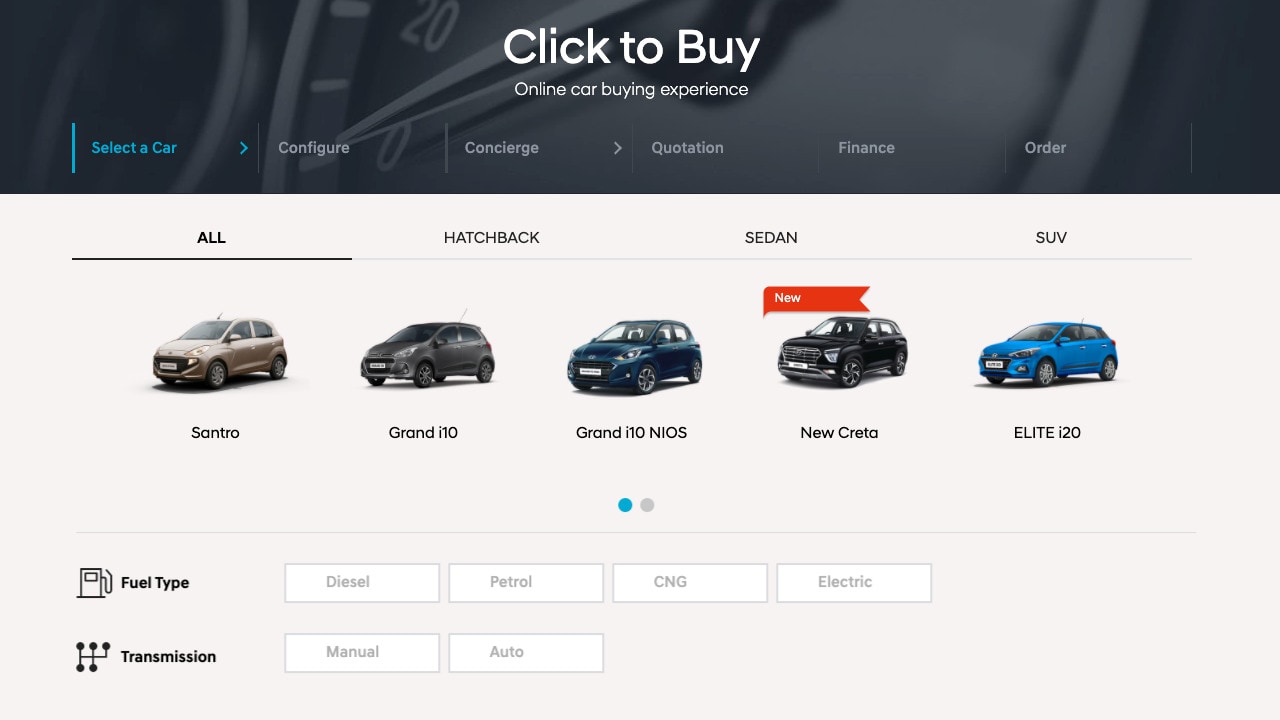The image features a centered white text that reads "Click to Buy" with the tagline "Online Car Buying Experience." The background showcases a speedometer, with the needle positioned at zero and the next marked line indicating 20. The entire background is rendered in shades of black and gray.

To the top left, the phrase "Select a Car" is highlighted in blue text, accompanied by a left-aligned line and a right-pointing arrow. Further across, the words "Configure," "Concierge," "Quotation," "Finance," and "Order" are displayed sequentially in white text, each separated by right-pointing arrows.

Beneath this section, in black text, the word "All" appears prominently underlined, followed by options "Hatchback," "Sedan," and "SUV." 

A series of small car images are aligned vertically:
1. A small gray car labeled "Santro" (S-A-N-T-R-O)
2. Another small gray car identified as "Grand i10"
3. A small blue car also labeled "Grand i10" alongside the tag "iOS"
4. A black car with a red "New" banner, captioned "New Creta" (C-R-E-T-A)
5. On the far right, a bright blue car labeled "Elite i20"

This visually rich composition effectively outlines a seamless online process for selecting and purchasing cars.